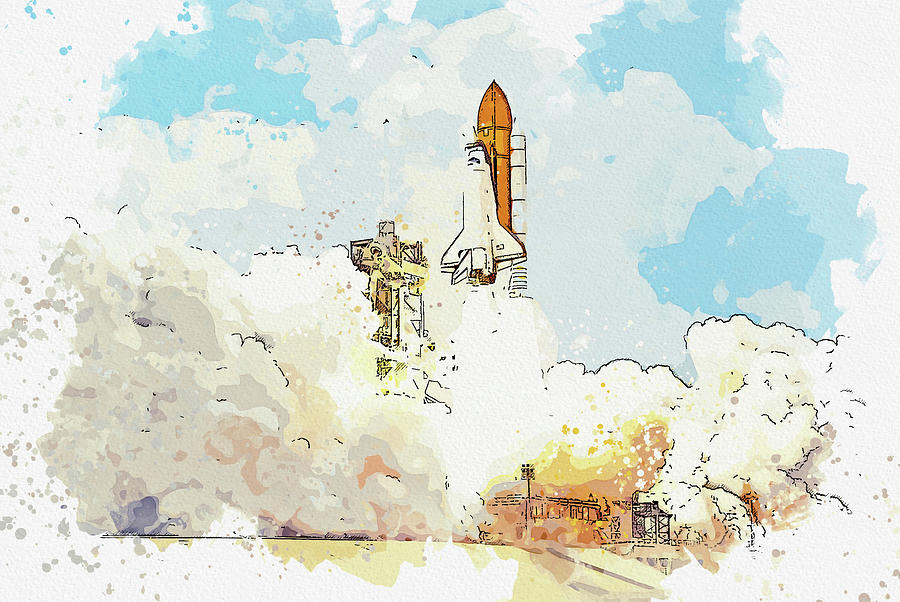This illustration, which appears to be a digital creation emulating a watercolor style, depicts a dynamic scene of a rocket launch. The focal point is a white rocket ship with black outlines, attached to an orange booster, ascending into the sky. Surrounding the rocket is a voluminous cloud of gray and white smoke, interspersed with fiery red and orange hues, signifying the intense heat and energy of the launch. The background showcases a hazy, light blue sky filled with scattered clouds, transitioning to a more vibrant and chaotic mix of grays, oranges, and tans towards the bottom, where hints of structures and buildings, partially obscured by the smoke, provide context and depth. The image's texture resembles watercolor paper, and the colors fill the space with a recognizable yet slightly abstract cartoony feel, emphasizing the illustration's artistic rather than photorealistic nature.